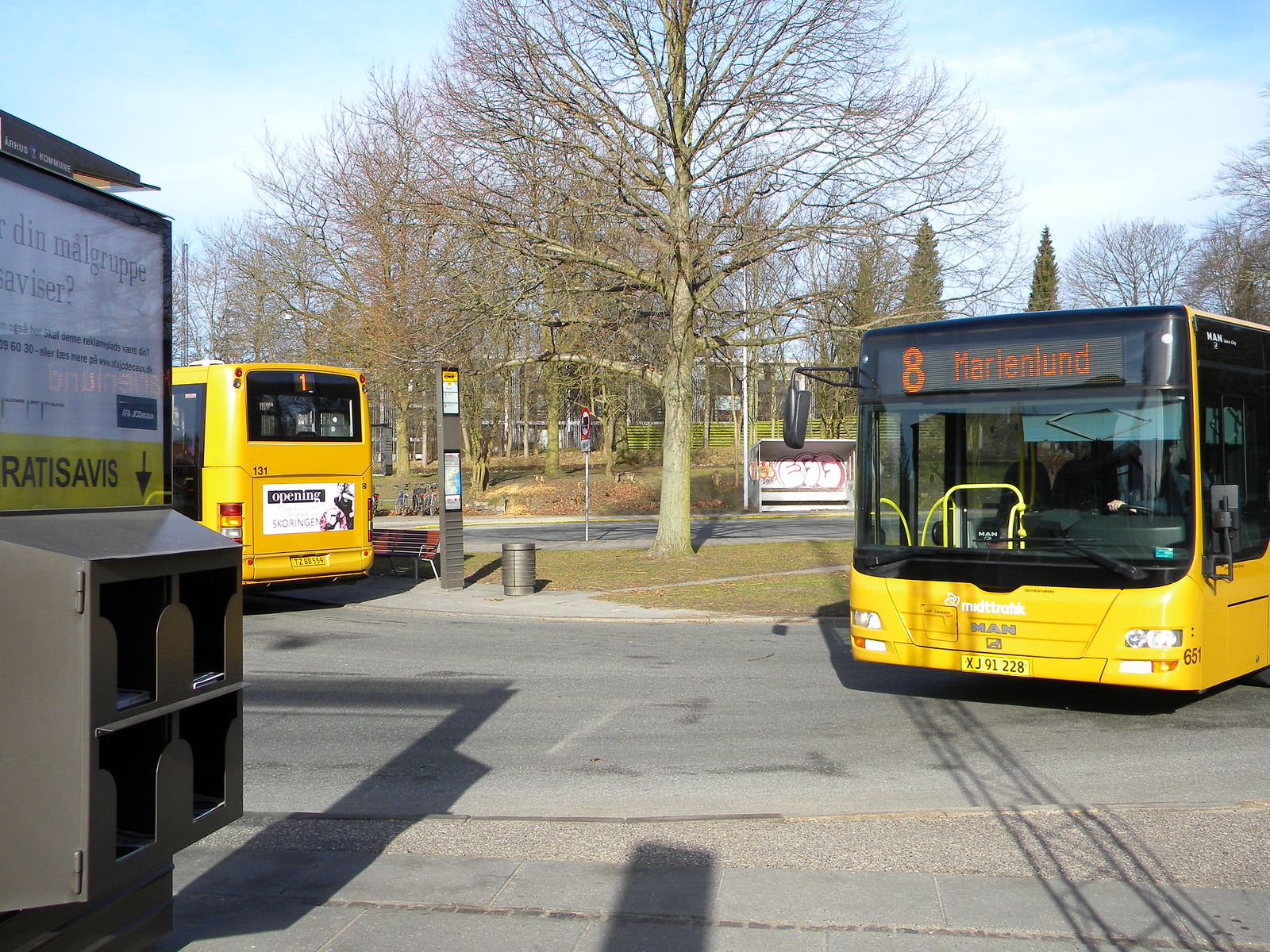The image depicts a busy bus depot or bus stop set against a light blue sky with a backdrop of trees. Central to the scene is a large, leafless tree, suggesting it might be a chilly day. To the right of the tree, a yellow bus numbered 8 and labeled "Marienlund" is turning into the street. The yellow bus features black windows and trim. To the left of the tree is a bus stop marked with a vertical signpost that possibly displays a map and timetable. Adjacent to the signpost, the back of another yellow bus numbered 1 is visible. This bus stop also features a wooden bench for waiting passengers, which shows signs of graffiti. The background further incorporates various signage intended to guide passengers. An advertisement is visible on the back of the departing bus, and the surroundings, filled with tree branches, indicate a park-like setting.